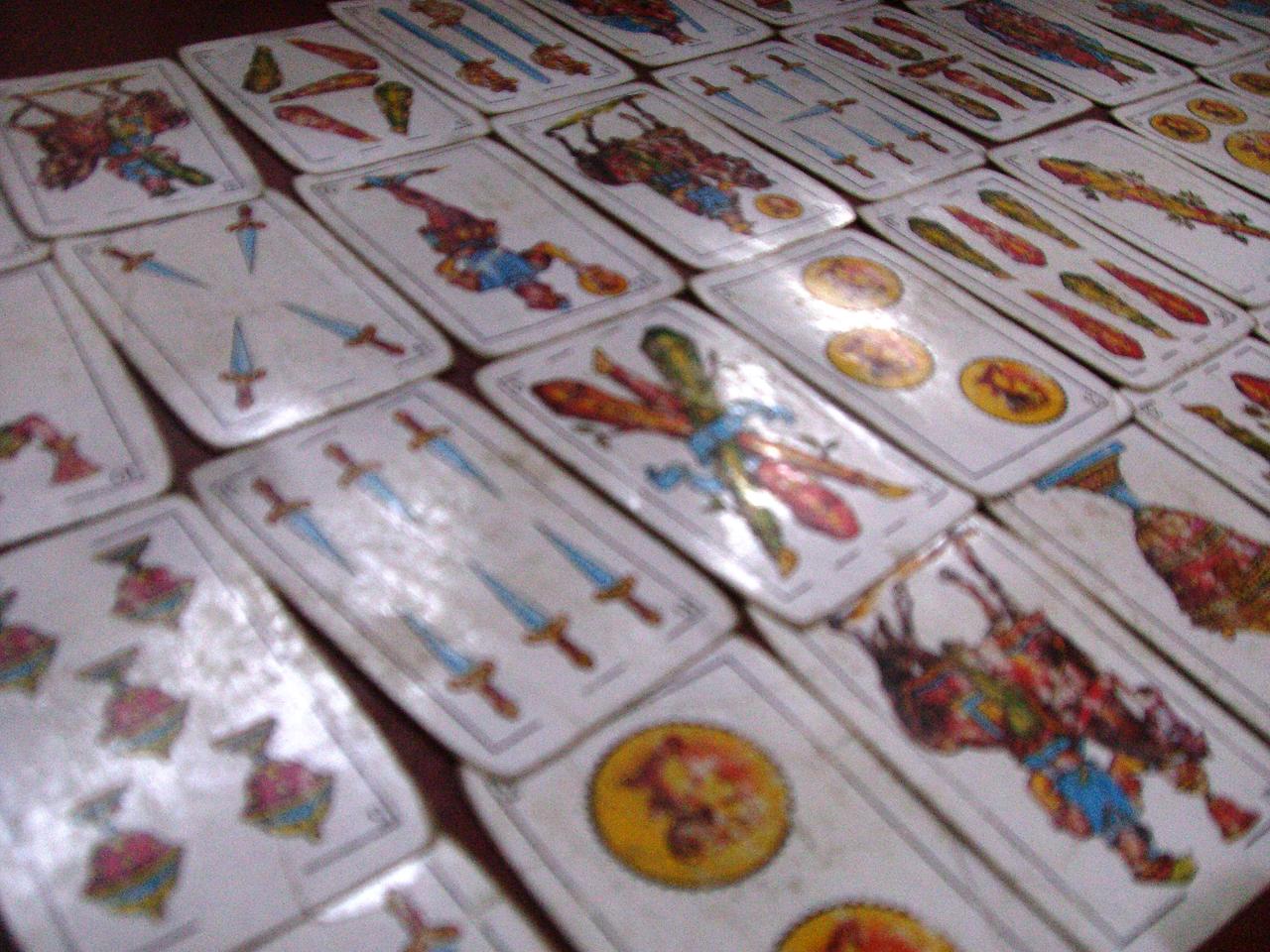The image depicts a sprawling tarot card deck meticulously laid out, showcasing a variety of intricate designs and symbols. Prominently featured among the spread are the Six of Swords and the Four of Swords, each with their unique, detailed artwork. The cards are scattered across a surface, creating an impression of a comprehensive reading in progress. When viewed in reverse, the tarot cards reveal their mirrored interpretations, adding to the depth and intrigue of the scene. This captivating display highlights the rich, esoteric tradition of tarot reading.